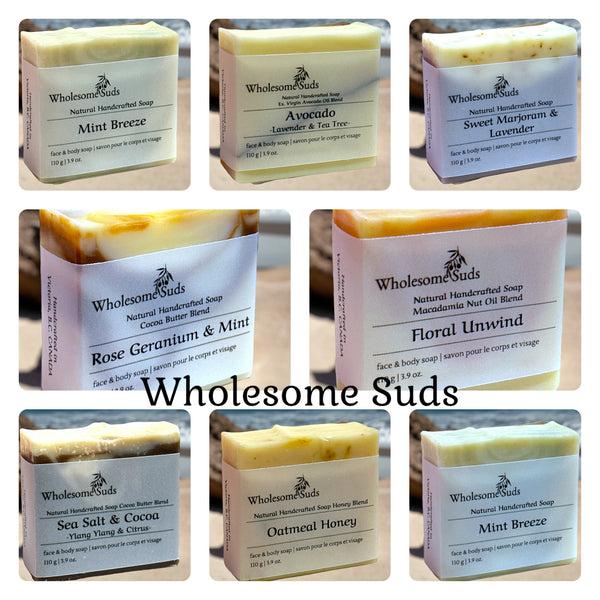This photo is an advertisement for the handmade soap brand Wholesome Suds, showcasing a colorful array of their artisanal products. The image features 8 distinct variations of the soap, each meticulously boxed and labeled with the brand’s logo and the text "Natural Handcrafted Soap, Cocoa Butter Blend, Face and Body Soap." The scents include Mint Breeze, Avocado, Sweet Marjoram and Lavender, Rose Geranium and Mint, Floral Unwind, Sea Salt and Cocoa, Oatmeal Honey, and another instance of Mint Breeze. The small, square soaps are wrapped in elegant white paper that highlights the product details and scent distinctions. The soaps present a mix of tan, white, and hints of orange hues, arranged neatly, making a visually appealing display likely aimed at social media or blog viewers. This high-quality image captures the artisanal and wholesome essence of the brand, which appears to be a small, independently owned business.